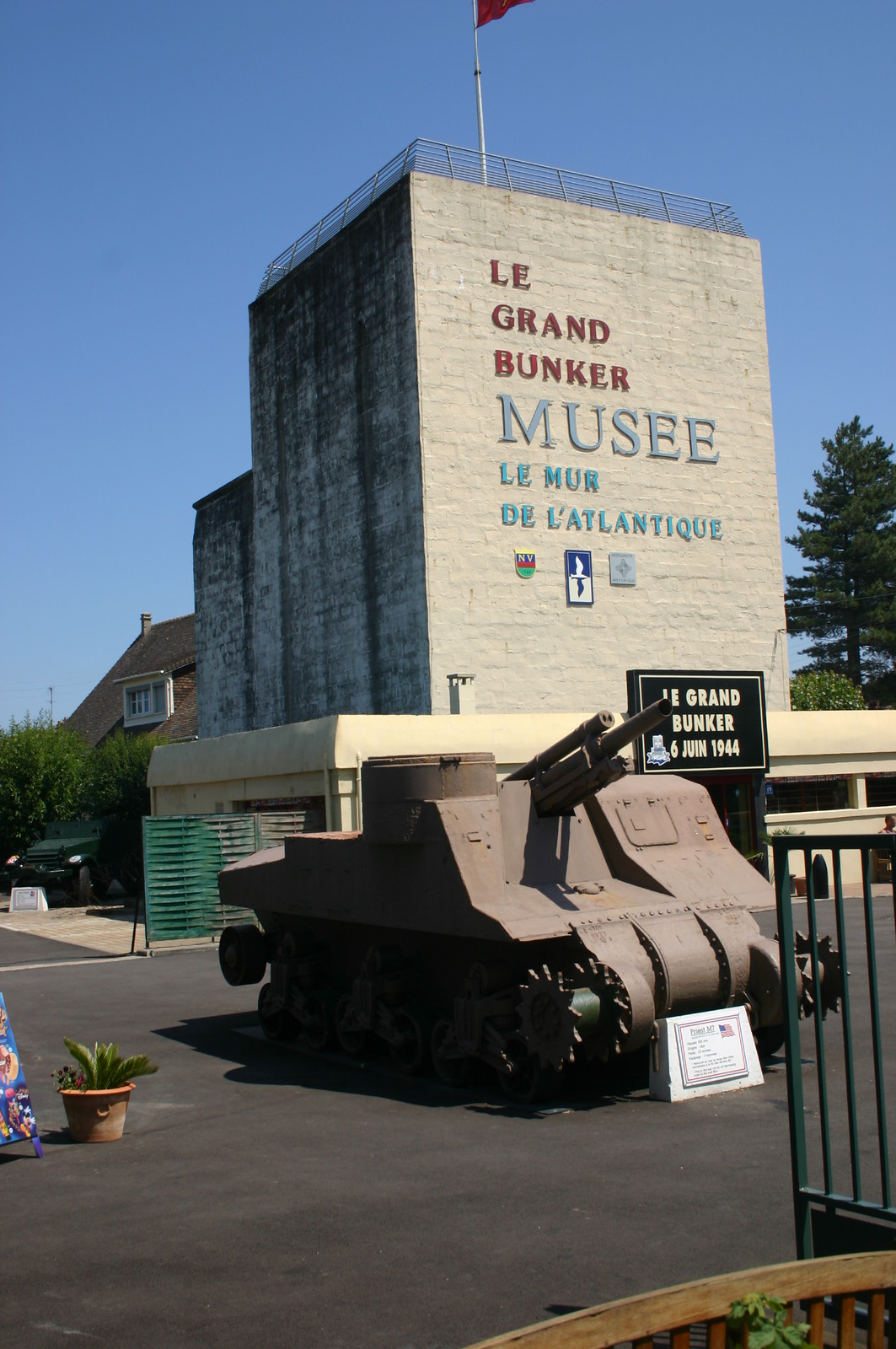This photograph depicts a small, rusted tank with a slight pinkish hue, positioned on a blacktopped platform outdoors. The tank appears to be very old and lacks treads, showcasing distinctive spiky star-shaped wheels. In front of it sits a white informational sign. The background features a large, aged, windowless building with dirty, light grey walls and a prominent brick tower. The building's façade bears the inscription "Le Grand Bunker Musée," indicating it is a military museum. The scene includes an entrance area akin to a parking lot or walkway, with trees and a nearby house visible in the distance, and a gated section to the right.